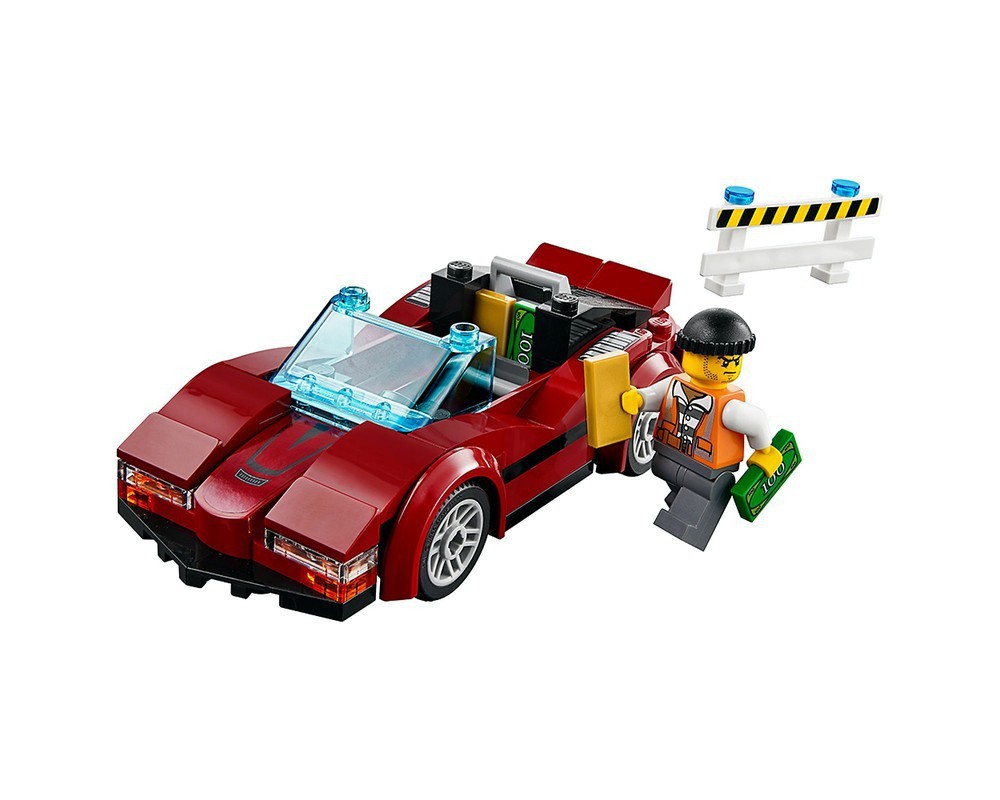In the center of a predominantly white background, a red Lego car and a Lego figurine are prominently displayed. The deep red car features a V-shaped gray logo on the front hood, a black underside, and a black stripe along its side door. It stands sturdy on black tires and has a translucent blue windshield. A battery pack is detailed in the back of the car. Beside the car stands a Lego man, predominantly yellow, wearing a black cap, an orange vest with white sleeves indicating construction gear, and gray pants. He holds a block of money labeled "100" in one hand and a golden block, likely resembling a gold bar, in the other. His face sports a mean expression, suggesting he might be a bank robber. Behind him is a white signpost with black and yellow stripes, topped with two blue knobs. The scene is detailed with additional elements like a translucent blue window in the red car and distinct construction-like accessories.